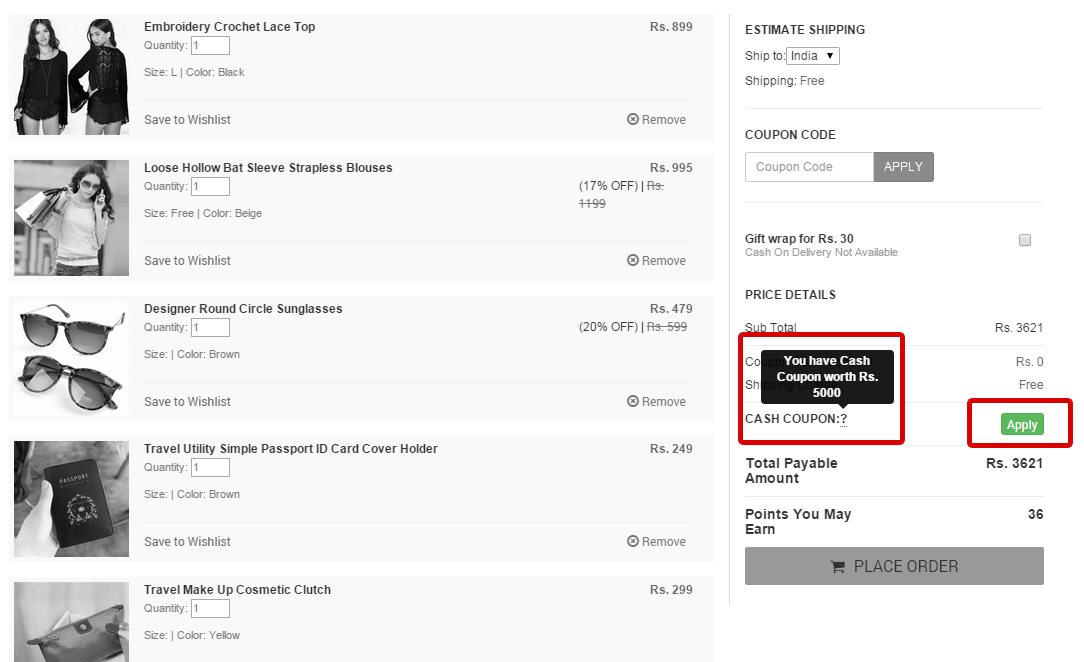This image appears to be a screenshot from an e-commerce website displaying a shopping cart summary with detailed descriptions of the items selected for purchase. The layout consists of a left column with product images and descriptions, and a right column featuring payment and shipping details.

In the upper left corner, there's an image of a woman dressed in a long black shirt paired with lacy shorts. Below this image, the product is described as "Embroidery Crochet Lace Top," with a quantity of one, size large, and color black, priced at RS-899.

The next item features a woman in a light-colored shirt holding a bag over her shoulder. She has long dark hair, wears sunglasses, and is talking on a cell phone. The product is listed as "Loose Hollow Bat-Sleeved Strapless Blouses," with a quantity of one in size free, and color beige, priced at RS-995.

Following this, there are two pairs of sunglasses labeled as "Designer Round Circle Sunglasses," with one pair selected in color brown, priced at RS-479.

A passport cover is also visible, described as "Travel Utility Simple Passport ID Card Cover Holder," with one item in color brown, priced at RS-249.

Additionally, there's a makeup pouch listed as "Travel Makeup Cosmetic Clutch," with one item priced at RS-299.

On the right side of the page, the payment area details include sections for estimated shipping, with India as the destination. There's also a field for entering a coupon code, which is currently blank. A significant red rectangle highlights a cash coupon worth RS-5000, and another red rectangle surrounds the green "Apply" button.

At the bottom, below the red rectangles, there's a "Place Order" button accompanied by a shopping cart icon, allowing the user to finalize their purchase by clicking it.